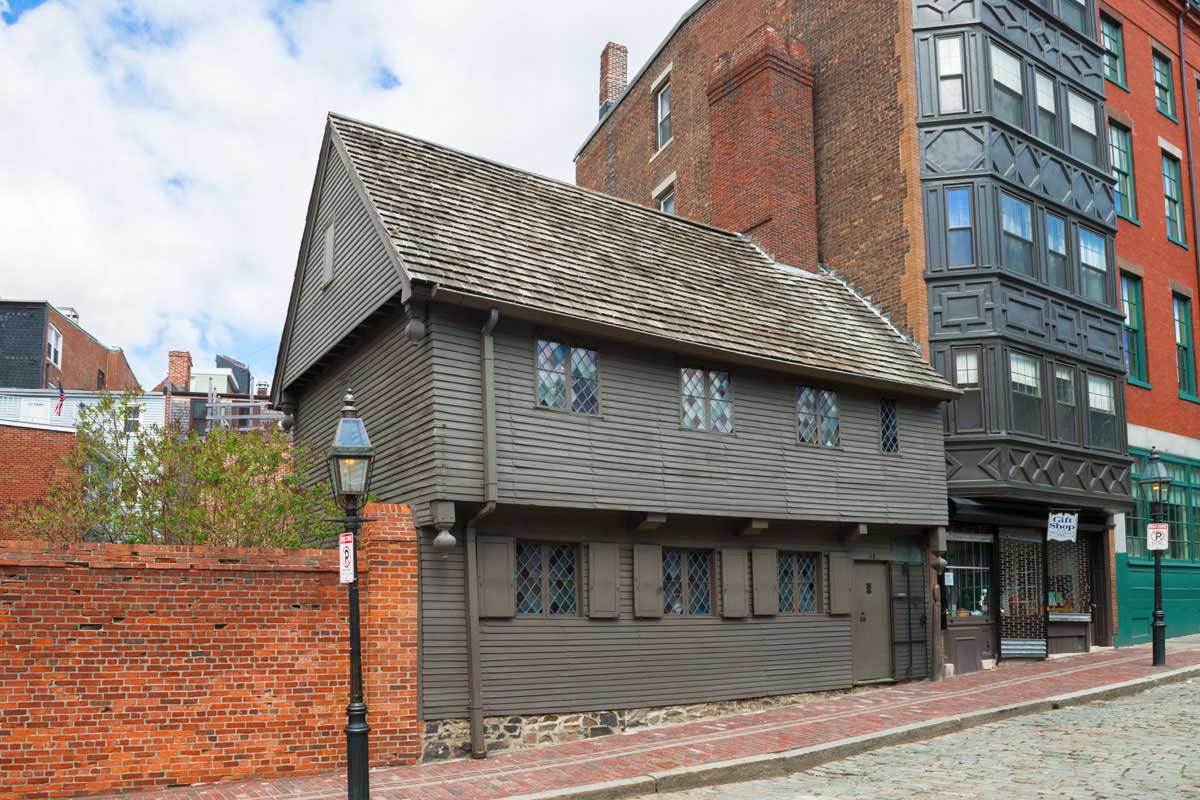This outdoor daytime photograph captures a quaint street scene with a charming assortment of buildings. On the left side of the image, a red brick wall partially obscures a small tree behind it. Adjacent to this wall stands a picturesque, brown, two-story building with an attic under a weathered brown roof, marked by brown and white streaks. The building's exterior is adorned with dark brown wooden panels and features brown shutters flanking the windows on the ground floor. Above a wooden door on the right side of this structure, a small window sits, matching the alignment of the three-over-three window design. A red brick chimney emerges from its roof, adding to its old-world charm. The street in front of these buildings is paved in brown cobblestones, complemented by a red brick sidewalk and black, old-fashioned streetlights.

To the right of this small house, a towering four or five-story building stands, likely a residence, with dark brown or black brick siding. This building seamlessly connects to another red brick structure of similar height, both touching without any gaps in between. Beyond these buildings, the scene hints at modern city structures in the distant left background. The entire setting is illuminated by a diffused, mostly cloudy sky, allowing only fleeting glimpses of blue amidst the puffy clouds.